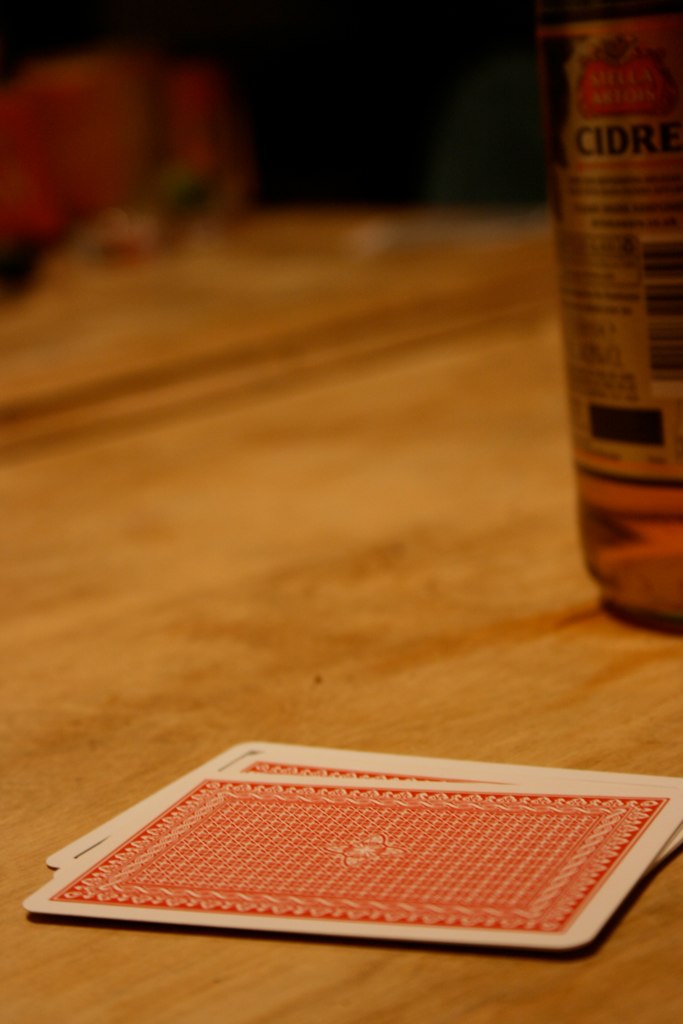In the photograph, a pair of playing cards are stacked face down on a light brown, unstained wooden table, capturing the eye as the most prominent feature. A portion of a blurry, balled-up hand is visible in the background on the top left, against a dark backdrop, making it difficult to identify clearly. On the right side of the image, a can labeled "cider" partially enters the frame but is cut off and blurred, making the additional text unreadable.